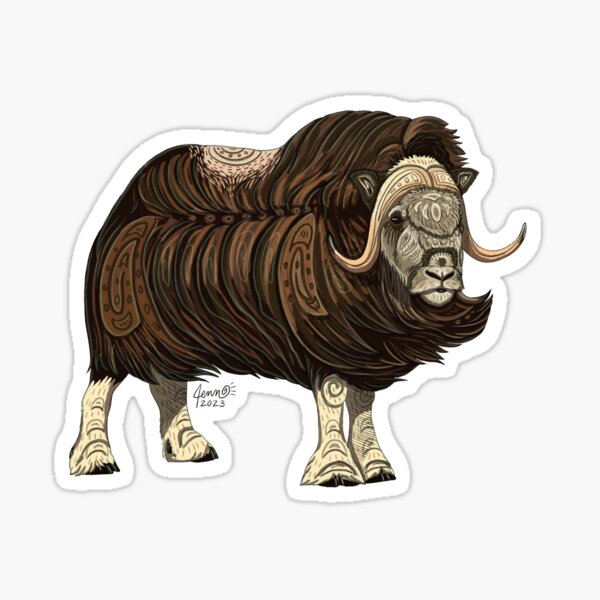The image depicts a detailed sticker or cut-out art of a bison with elaborate and ornate markings. The bison's body is covered in dense dark brown fur adorned with intricate patterns, suggesting that some parts might have been artistically shaved or designed to showcase these images. The bison's head, facing right, is grayish off-white, matching the color of its legs. Its stance is on all fours, with the front legs together and the back legs spread apart. Various markings can be seen on its fur, head, and horns, including circular and dotted patterns. Beneath the belly of the bison, next to the back legs, there is a signature in cursive reading "Gemma 2023." The entire artwork is affixed to a white-colored platform, with the bison positioned at a slight angle that clearly displays its side profile and all four legs. The blend of earthy tones such as brown, tan, beige, and black lends a realistic yet artistic touch to the piece.